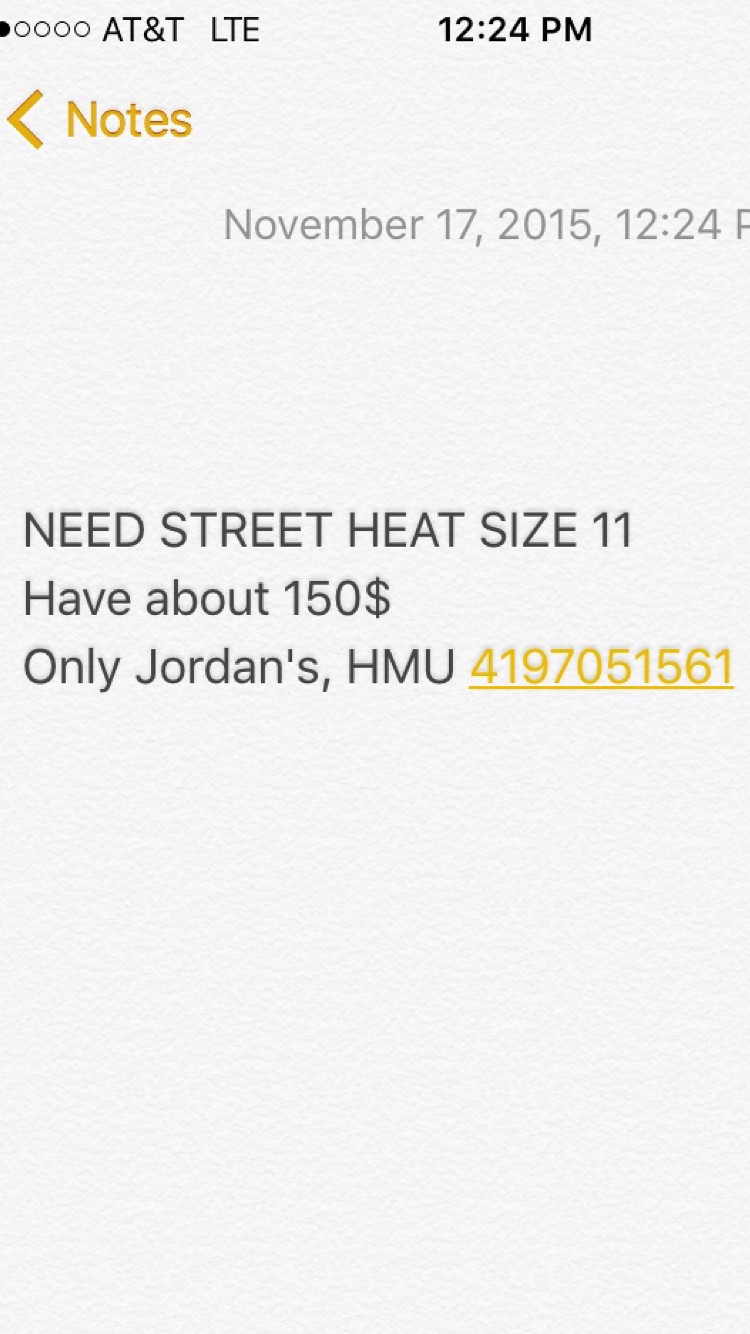The image is a screenshot of an iPhone on the AT&T LTE network, taken at 12:24 p.m. on November 17, 2015. The screen displays a "Notes" app with a note that reads: "Neat Street heat size 11 have about $150 only Jordans, HMU" followed by the contact number "419-705-1561." The background of the note is off-white or gray, while the rest of the screen is completely black, except for the displayed text.